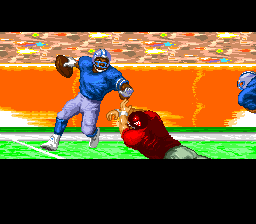A screenshot captures a small square image from a retro-style video game, depicting a dynamic football scene. In the forefront, a player in a blue uniform, complete with a blue and gray helmet, white-accented sleeves, and white shoes, clutches the football as he maneuvers on the green and white field. Opposing him is a player donning a red uniform and white pants, positioned to block with his hands outstretched. An orange banner with white streaks stretches across the background, adding to the vibrant atmosphere. To the right of the action, another player stands poised, while the stands are filled with fans, represented as brown and yellow blobs, cheering the players on.